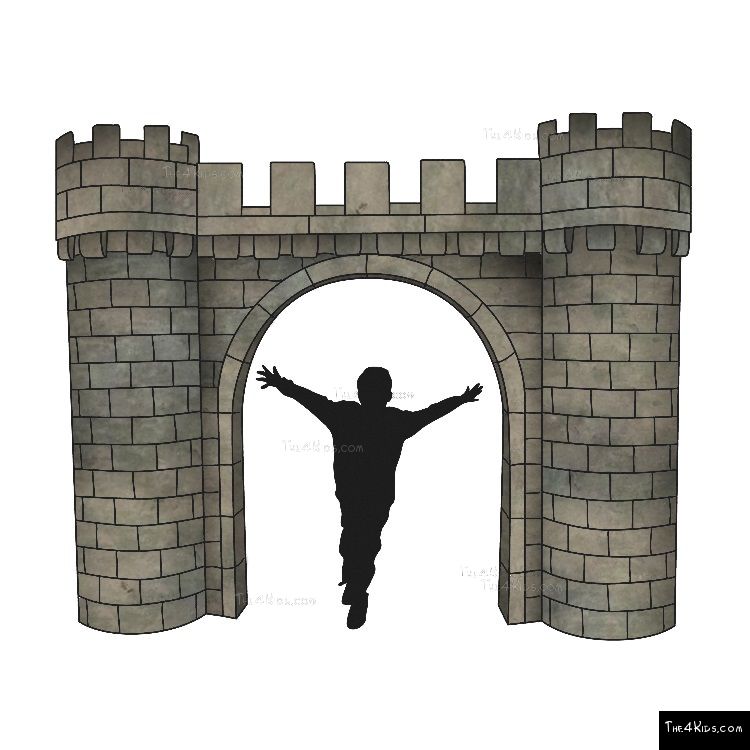The image is a cartoon-like drawing of a silhouetted young boy walking through an archway of a castle. The boy, positioned center screen, stands beneath a stone archway, raising one arm, seemingly trying to touch the sides of the arch. The castle, drawn in a playful, child-friendly style, features cylindrical towers capped with crenellated tops, resembling the classic castle crown. The structure is depicted with grayish-brown bricks outlined with black mortar lines, enhancing its hand-drawn appearance. Surrounding the central archway, additional brickwork and towers flank the scene, contributing to the castle-like atmosphere. On the bottom right of the image is a black box with white text in a handwritten style, reading "time4kids.com," set against a white background.